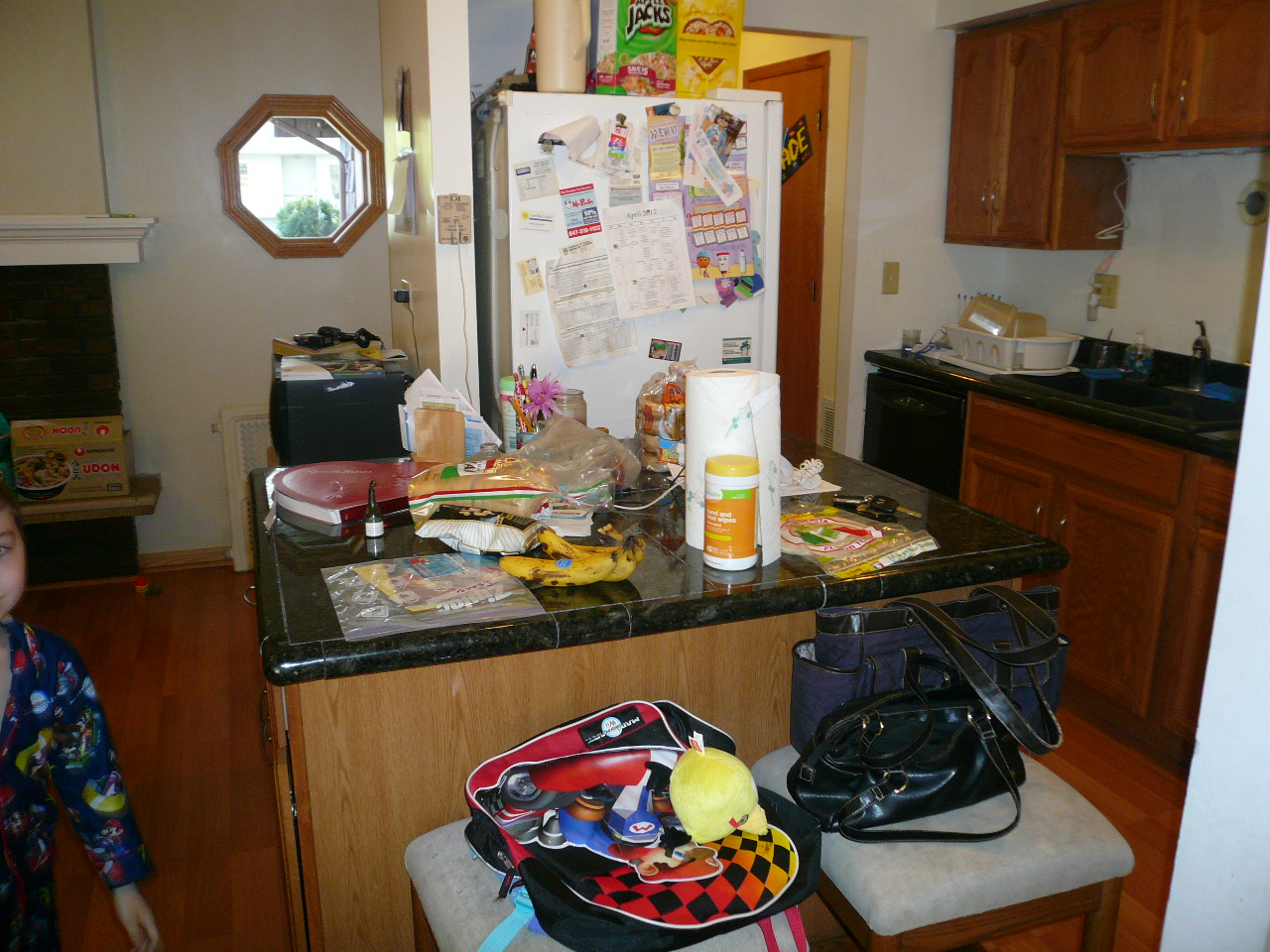This indoor photograph captures a cozy kitchen scene. On the left, a young child in colorful Super Mario Bros. pajamas is partially visible. The kitchen table is cluttered with various items including car keys, overripe bananas, a Ziploc plastic bag, sunflower tortillas, a roll of paper towels, a bag, Valentine's candies, a red heart, a loaf of bread, a bag of popcorn, a candle, multiple pens and pencils. The refrigerator in the background is adorned with several papers, and its top is stocked with boxes of Apple Jacks and Cheerios cereal.